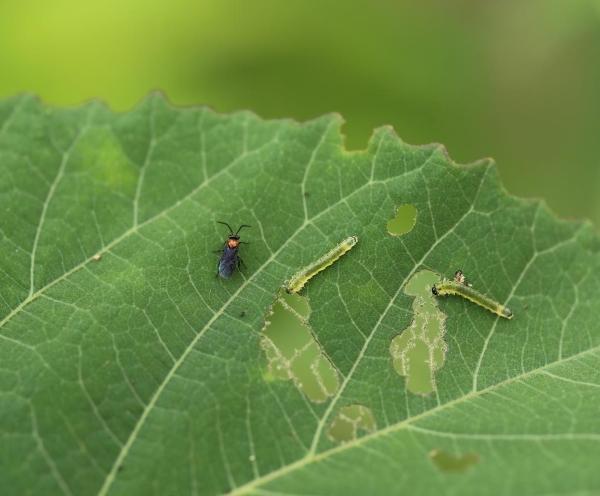The photograph is a close-up image of a green leaf, with a blurred, greenish background. Dominating the scene is the leaf, upon which three insects reside. Two of these insects are translucent green worms, or caterpillars, about half an inch long, and possibly fuzzy, with black tips at their heads. These caterpillars are actively eating the leaf, evidenced by several large, discolored holes. Positioned near the center of the leaf is a small, purplish-black beetle-like insect with antennas and six legs, approximately three-quarters the size of the caterpillars but thicker in build. The overall health of the leaf appears poor due to the feeding insects.